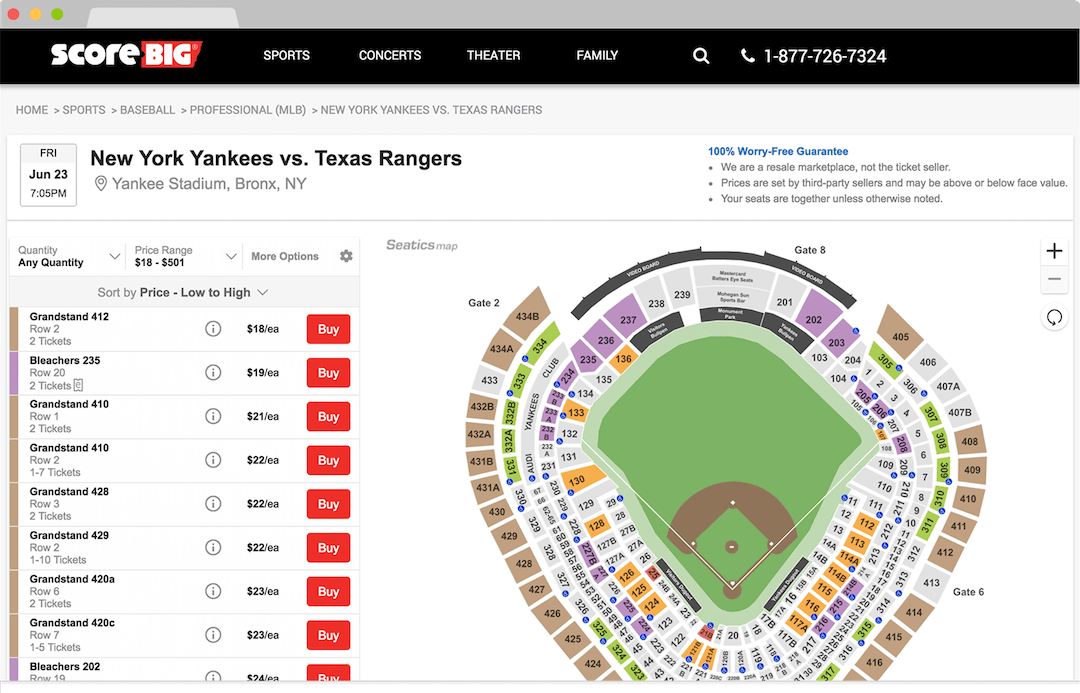Screenshot of a ticket purchasing website for a baseball game at a stadium. The top portion features a gray border with red, yellow, and green dots in the upper left-hand corner. Below, a black banner with bold white text reads "Score Big," where "Big" is emphasized on a red background. This section also includes navigation options in white text: "Sports," "Concerts," "Theater," "Family," along with a magnifying glass icon for searching, and a phone number: 1-877-726-7324.

The header displays breadcrumbs showing "Home > Sports > Baseball > Professional MLB > New York Yankees vs. Texas Rangers," indicating the game the user is interested in. The details of the game are listed as "Friday, June 23rd, 7:05 p.m."

To the right, there is a message saying, "100% worry-free guarantee. We are a resale market, not a ticket seller. Prices are set by third-party sellers and may be above or below face value. Your seats are together unless otherwise noted."

Below, a map of the stadium showcases numbered sections. Ticket options available show a quantity of any and a price range from $18 to $501, with more filtering options including sorting by "Price low to high."

Displayed ticket prices range from $18 to $24 each, covering various stadium sections: Grandstand 412, Bleachers 235, Grandstand 410, Grandstand 428, Grandstand 429, Grandstand 420A, Grandstand 420C, and Bleachers 202.